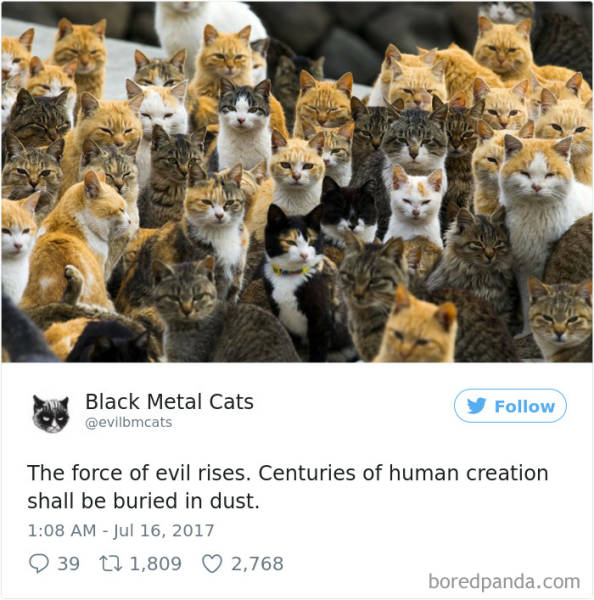The image is a social media post from Twitter, dated 1:08 AM, July 16, 2017, and features a mass gathering of approximately 25 to 30 cats of various colors, including brownish-gray, orange with white, calico, and tabby with white. All the cats are closely packed together, sitting or standing, and staring straight at the camera with squinty eyes. Notably, there are black and white cats in the center and slightly blurred larger white cat towards the left background. The scene appears chaotic yet organized, with every feline facing forward, creating an almost surreal visual. The bottom left corner displays a logo of a cat head next to the text "Black Metal Cats" followed by the handle "@evilBMcats." To the right is a blue "Follow" button with the Twitter bird icon. Below the image, it reads, "The force of evil rises, centuries of human creation shall be buried in dust." The post has accumulated 2,768 hearts, 1,809 retweets, and received 39 comments. The lower right-hand corner marks the post as originating from BoredPanda.com.